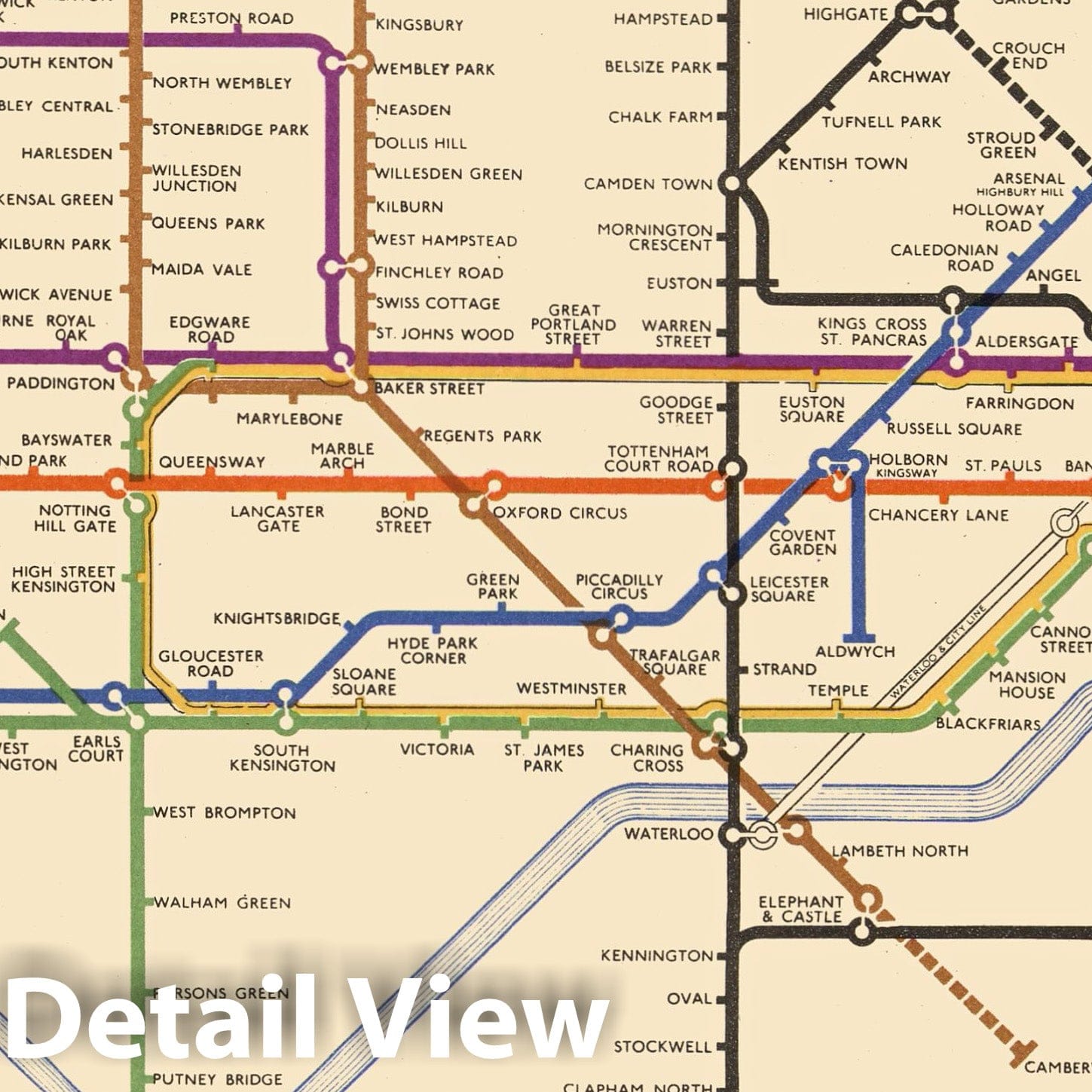The image appears to be an old, detailed map of London's subway system, prominently featuring various lines in distinct colors including brown, blue, green, orange, purple, black, and yellow-brown. The map boasts a beige background with "Detail View" written in large white letters with a shadow effect in the bottom left corner. This particular map offers a plethora of location names, such as Putney Bridge, Willesden Green, West Brompton, Victoria, Aldwych, Chancery Lane, and Goodge Street, among others. Numerous colored lines create patterns and diagonal routes indicating connections to various parts of the city, such as Baker Street, Kilburn, Neasden, Kingsbury, North Wembley, and Stonebridge Park. Additionally, a waterway, identifiable by thin blue lines labeled Waterloo, runs through part of the map. Overall, the map serves as a historical guide to navigate London's extensive subway network.